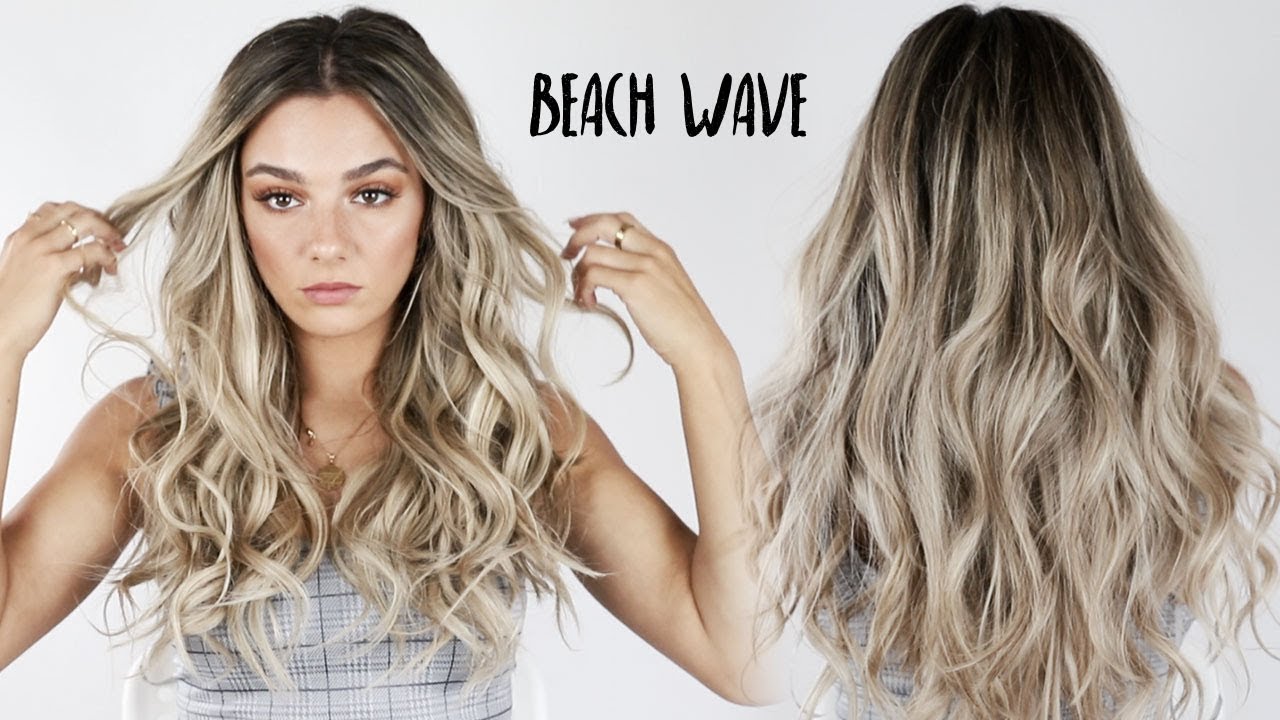The image presents a detailed view of a woman’s hair in a dual photograph layout against a gray background, with the caption "Beach Wave" in a trendy font at the top center. On the left, the woman faces the camera directly, allowing a clear view of her long, wavy hair, which transitions from dark roots to bleached blonde tips. She is dressed in a gray plaid shirt with white and black stripes, accessorized with gold rings and a gold necklace. Her makeup is elaborate, highlighting her tan complexion. She holds strands of her hair in both hands, bringing them over her shoulders, emphasizing the hair’s length and wavy texture that extends over her breasts. On the right, the back view of her hair is showcased, falling down to her mid-back and displaying the wavy pattern and highlights more prominently. The overall image accentuates the beachy, layered waves of her hair, styled to look naturally tousled and voluminous.